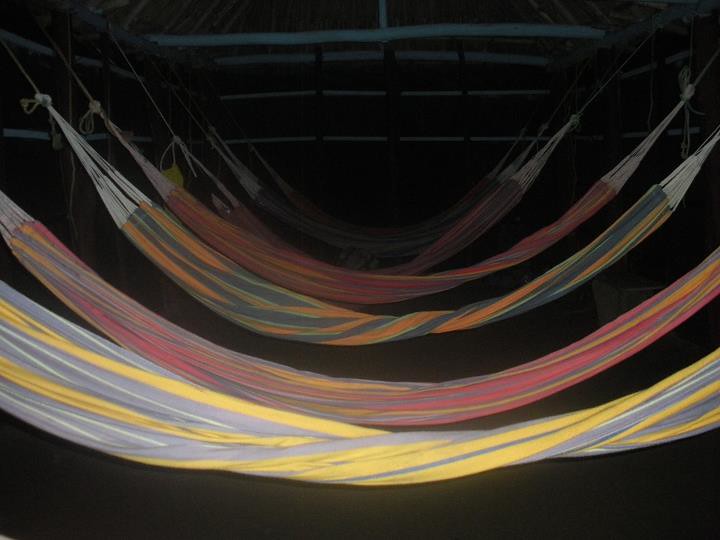In this detailed and dark image, we see a horizontal row of seven or eight hammocks hanging within what appears to be a dimly lit warehouse or garage. The backdrop is predominantly black, adding to the obscurity of the scene. At the top of the image, there are a few light gray bars, possibly serving as structural elements to which the hammocks are attached. The hammocks themselves are vividly colorful and striped: the first hammock features light purple, blue, and yellow stripes with thin white lines; the second hammock displays a mix of red, purple, and yellow colors; the third hammock has dark gray and orange stripes. The fourth hammock resembles the second with its rainbow-like colors, while the remaining hammocks are too enshrouded in darkness to distinguish their hues. Each hammock is tied to poles with visible ties at both ends, and there is a hint of possible windows or skylights near the upper part of the building, casting faint light into this otherwise shadowy scene.